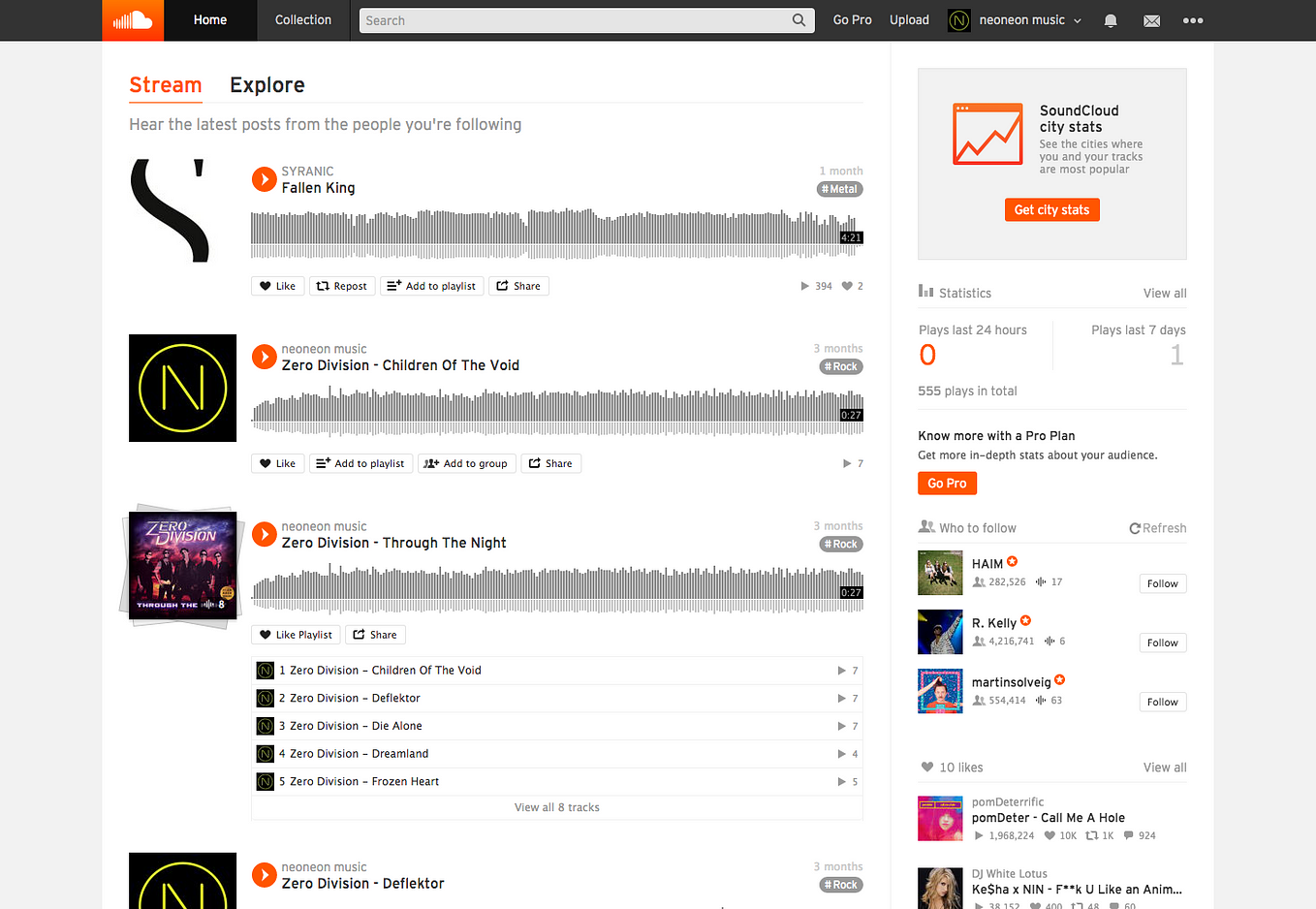This detailed description of the SoundCloud interface includes specifics about the web elements and the content displayed, providing a thorough overview of the layout and functionalities:

---

The screenshot showcases the main section of the SoundCloud website. At the top, the recognizable cloud logo is visible alongside the 'Home' section. Next to it are various features including 'Collection,' a search box, 'Go Pro,' and 'Upload.' The user's profile name, 'Neon Music,' is shown with a small bell icon for notifications and a mail icon for messages.

In the central part of the interface, the 'Stream' and 'Explore' tabs are prominently displayed, allowing users to listen to the latest posts from accounts they are following. The first song listed is "The Fallen King" by Seranic, categorized under metal music, with options to like, add to a playlist, and view the song's 4:21 duration. A visual volume meter is also indicated.

Below this track are songs by Zero Division, including "Children of the Void," which features an 'N' logo, and another song titled "Through the Night." The left sidebar displays the corresponding album cover and what appears to be a playlist, listing tracks such as "Children of the Void," "Deflector," "Die Alone," "Dreamland," and "Frozen Heart." 

Towards the right upper corner, the SoundCloud city stats are visible, displaying the number of plays in the last hour, with the current count at zero. Below this, information about the Pro plan and suggestions on who to follow, including accounts like Haim, R. Kelly, and Martin Solveig, is provided. Finally, there are mentions of Pom Deeter and KeshaXN at the bottom of the list.

---